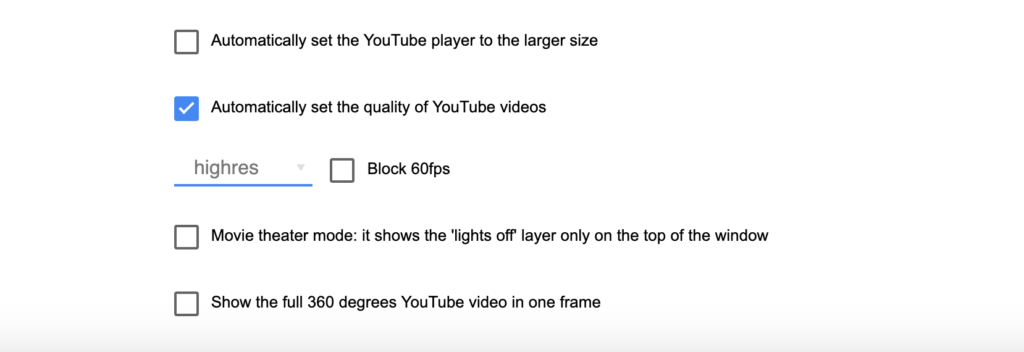Here is a cleaned and detailed caption for the image:

---

The screenshot is a small snippet taken from within a YouTube settings interface, set against a white background. In the top-left corner, there is an unselected, gray-colored square checkbox. To its right, in bold black text, it reads, "Automatically set the YouTube player to the larger size."

Below this setting, there is a blue box with a white checkmark inside it. Adjacent to it, in bold text, it states, "Automatically set the quality of YouTube videos." Continuing downward to the left, there is a blue horizontal line, with the word "High-res" written in gray lettering above it.

To the right of this blue line, there is an outlined, white square checkbox that is also not selected. Next to it, the text reads, "Block 60 FPS." Further below, there are two more entries, each featuring an unselected checkbox with a white-gray outline to their left. For the first checkbox on the right, the text reads, "Movie theater mode," followed by a description indicating that this option shows the lights off layer only at the top of the window.

The subsequent line, also in bold, states, "Show the full 360 degrees YouTube video in one frame." At the very bottom of the screenshot, there is a slight color transition where the off-white background changes to a pure white background.

---

This caption meticulously describes all the elements visible in the screenshot, providing a clear understanding of the YouTube settings depicted.